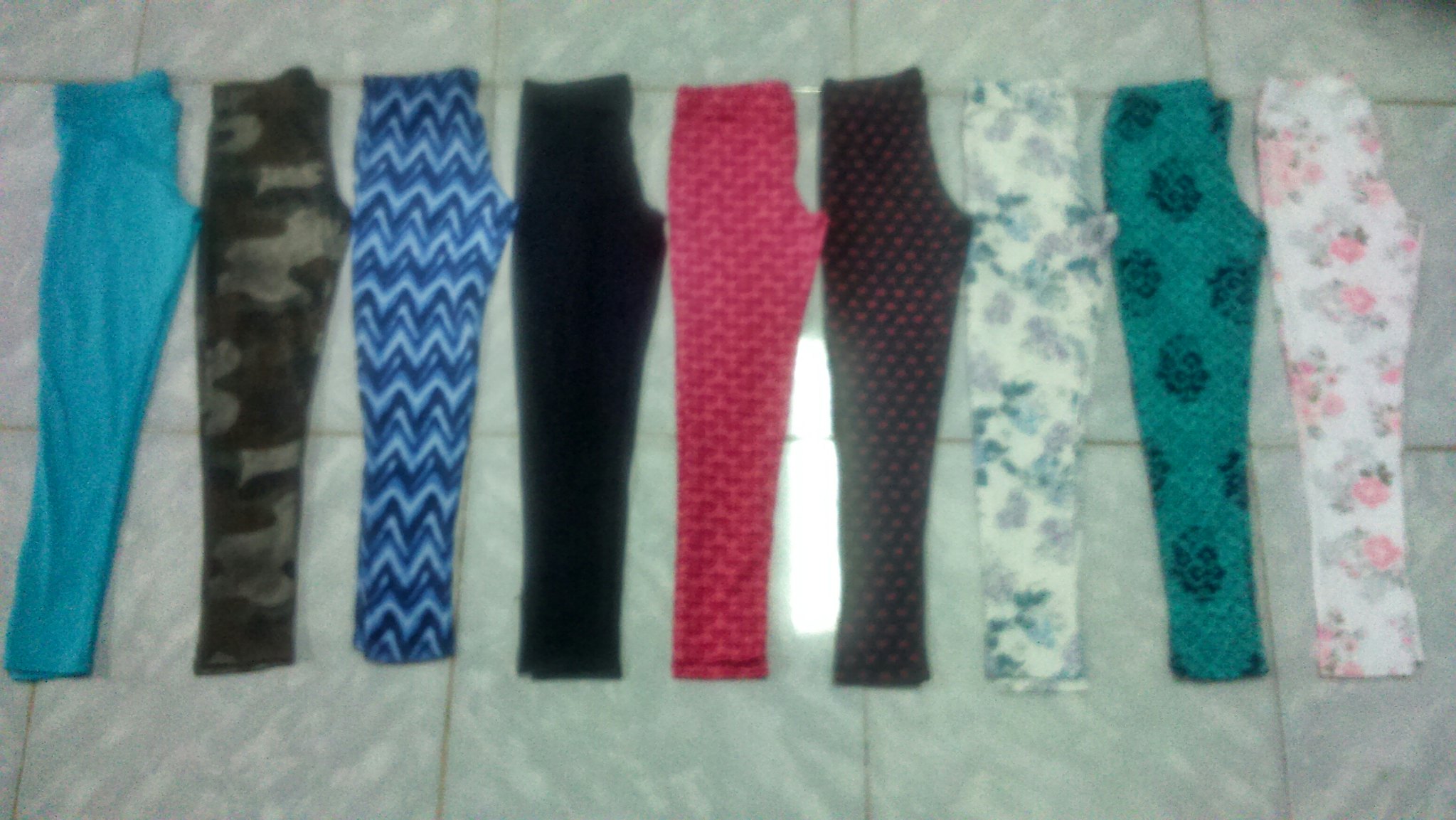The photograph showcases nine pairs of women's leggings neatly folded and arranged vertically on a gray and white tiled floor with tan grout. The layout reveals varying colors and intricate patterns, presenting a diverse collection. From left to right, the leggings are described as follows: a solid bright blue pair, a green camouflage design, a chevron pattern mixing light and dark blue, a plain black pair, a vibrant hot pink and red brick-like design, a primarily black pair adorned with alternating red polka dots, a white pair featuring blue-green leaves and lavender flowers, a tealy blue-green pair with black floral and diamond patterns, and finally, a pair with a white background decorated with light green leaves and baby pink flowers. The floor’s reflective surface and the somewhat blurry and possibly aged nature of the photograph add to the overall aesthetic of the image.